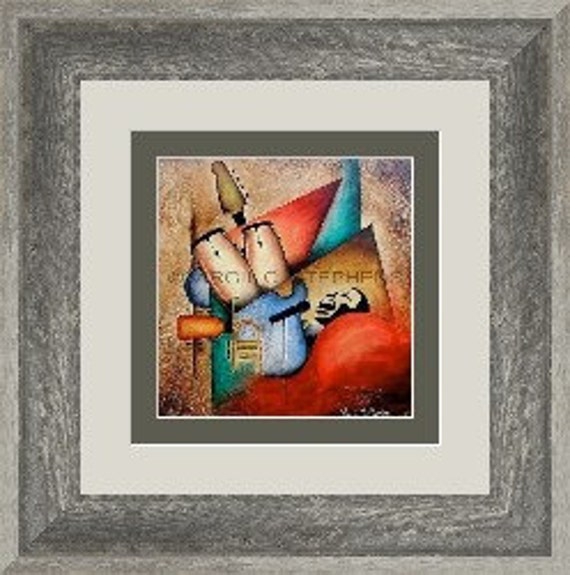The image is a framed print with a square, gray rustic wooden frame. Inside the frame, there are two mats: the outer one is white, and the inner one is a beveled gray. The print itself features an abstract, multi-colored painting with no discernible pattern, incorporating a variety of shapes and colors, including red, gold, blue, light brown, and orange. Central to the abstract imagery is the neck and body of a guitar, two bongos, and the face of a black man gazing upwards. Additionally, two corkscrew-like shapes, arches, and blobs of bright colors add to the complexity of the composition. The background color of the painting appears to be a sparkled light gold, almost bronze. There is a watermark across the front of the image, though it is illegible, and a possible artist's signature in the lower right-hand corner.